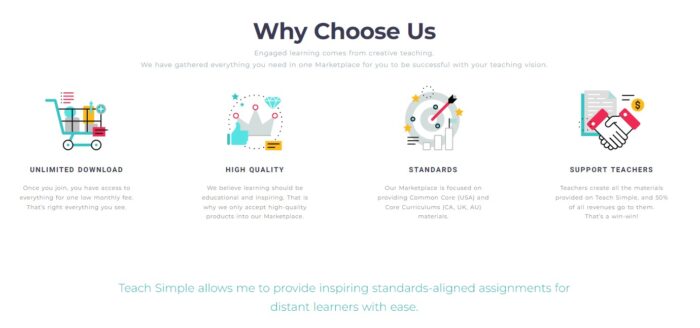This is a detailed screen capture of a website designed for educators. At the top of the screen, there's a prominent black title stating, "Why Choose Us." Beneath it, in gray text, is the slogan, "Engaged Learning comes from Creative Teaching." The description elaborates, "We have gathered everything you need in one marketplace for you to be successful with your teaching vision."

At the very bottom of the page, a light green testimonial reads, "Teach Simple allows me to provide inspiring standards-aligned assignments for distant learners with ease."

The central portion of the screen features four key icons, each accompanied by a description:

1. **Unlimited Downloads**: Represented by a shopping cart overflowing with items, it states, "Once you join, you have access to everything for one monthly fee. That's right, everything you see."

2. **High Quality**: Illustrated with a crown, a thumbs-up sign, and diamonds, this section highlights the platform's commitment to excellence: "We believe learning should be educational and inspiring. That is why we accept only high-quality products in our marketplace."

3. **Standards Aligned**: Depicted with a dartboard icon, it explains, "Our marketplace is focused on providing materials aligned with Common Core standards for the USA, Iceland, UK, and Australia."

4. **Support Teachers**: Featuring a handshake icon with a notepad behind it, this section emphasizes community support: "Teachers create all the materials provided on Teach Simple, and 50% of all revenue goes to them. That's a win-win."

Overall, the website positions itself as a comprehensive, quality-driven, and community-focused resource for educators seeking to enhance their teaching with minimal effort.